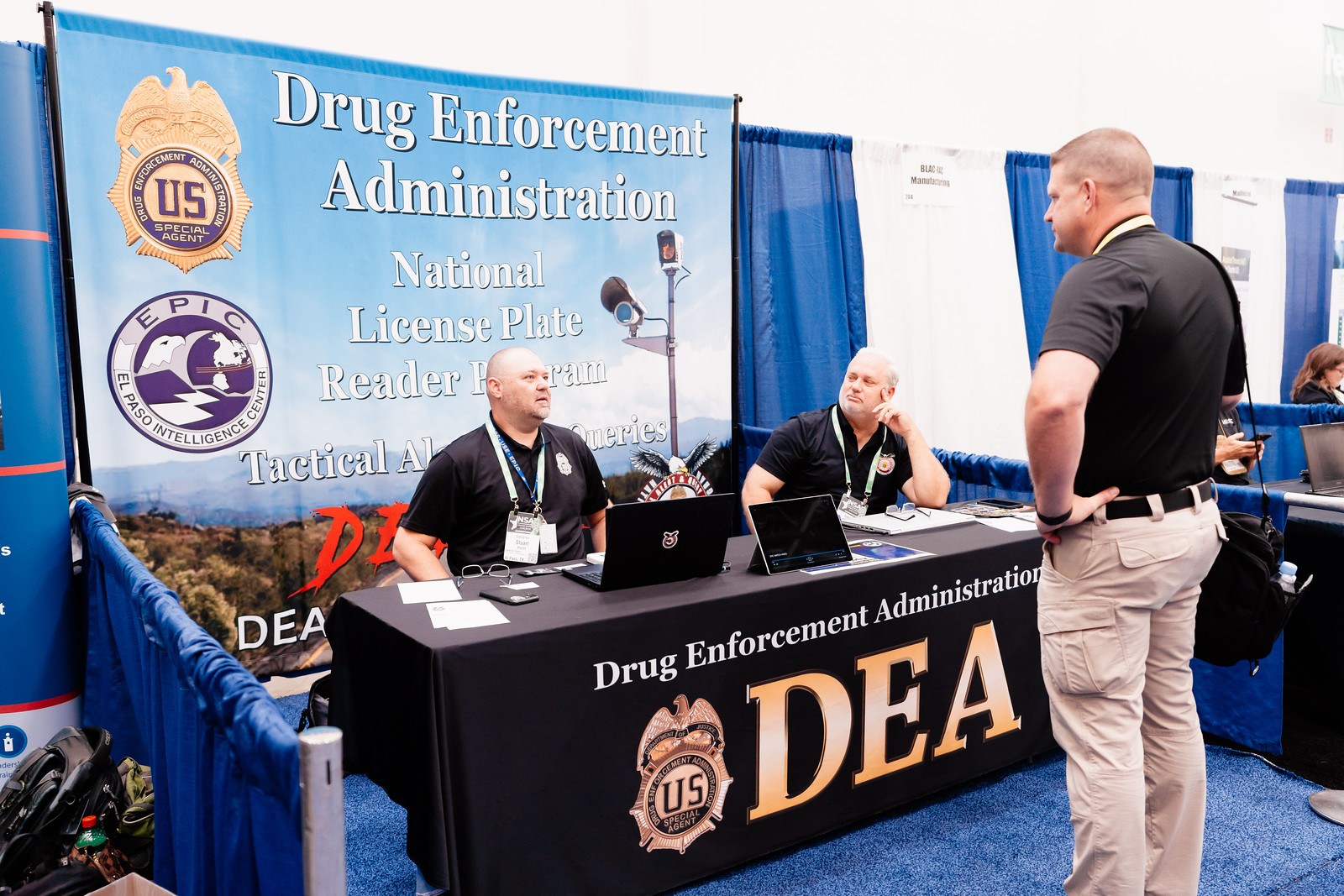The image depicts a bustling trade show or convention setting, featuring a prominent booth for the Drug Enforcement Administration (DEA). Sitting behind a black tablecloth that is emblazoned with the DEA acronym, the official US seal, and the words "Drug Enforcement Administration" in a gold, shiny font, are two large men dressed in black t-shirts. They are hunched over a laptop and an outwardly displayed iPad, engrossed in conversation with another man who stands to the right, dressed in a black t-shirt, khaki pants, and a black shoulder bag.

Directly behind the seated men is a large, eye-catching banner that announces the "Drug Enforcement Administration National License Plate Reader Program." The banner also includes additional, partially obscured text that suggests its association with tactical queries, and is adorned with a traffic camera image and the DEA badge. There's also an emblem for the El Paso Intelligence Center (EPIC).

The floor is carpeted, and the overall indoor setting is illuminated by conference or trade show lighting, with various hues of white, blue, gold, yellow, purple, tan, red, black, and white visible throughout the scene. The photo captures the moment against a backdrop of lively engagement, showing the DEA's outreach efforts in real-time.